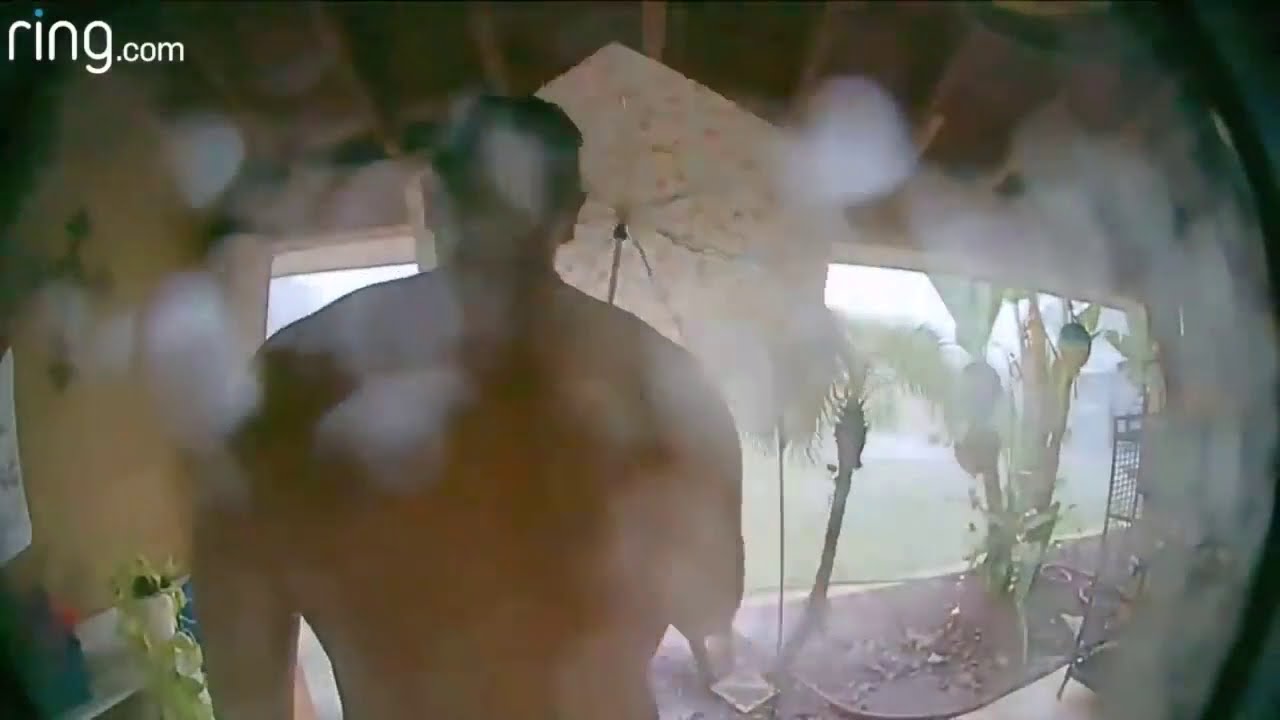In this image captured by a Ring video doorbell, evident from the "ring.com" logo in the top left corner, a shirtless and muscular Caucasian man with short hair stands prominently in the center left of the frame. The lens is smudged with water droplets, suggesting it's raining heavily, potentially during a storm or hurricane. The man, who appears to be on a porch or garage, holds an askew beach-style umbrella open in his right hand, seemingly battling the elements. Behind him, visible through the fisheye-distorted and rain-obscured lens, are small palm trees, a garden bed, and a large grassy lawn. The overcast sky and heavy rain further emphasize the intensity of the storm. The structure around him, with its wood-look ceiling, and a birdcage to the right, frames the chaotic outdoor scene.